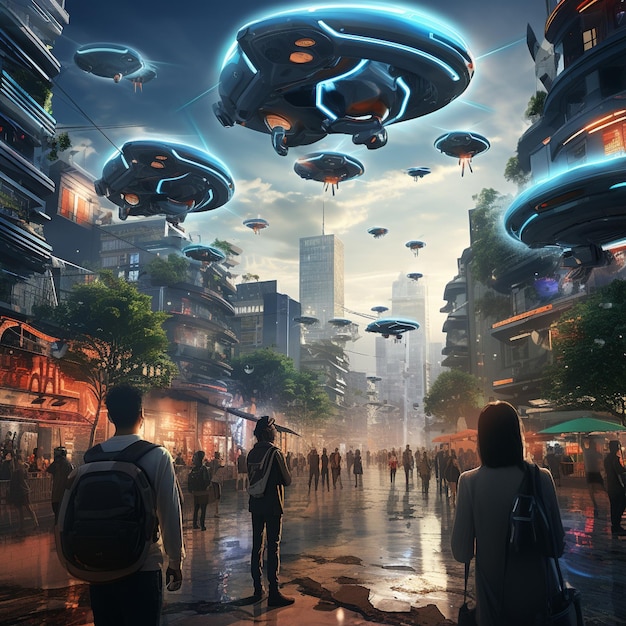In this vivid and detailed piece of futuristic artwork, a bustling downtown cityscape is depicted under an ominous, almost neon sky. The setting features towering skyscrapers and apartment buildings illuminated by a gradient of lightning blue, neon blue, and vibrant orange hues, imitating futuristic city lights. The focal point is a multitude of people standing on the busy streets and sidewalks, numbering around fifty, all gazing upwards in awe and curiosity at the spectacle above them. 

Hovering in the sky are about a dozen blue-colored spacecraft adorned with orange lights, emitting various beams and lasers that add to the tense and electric atmosphere. The buildings rise high in the background, some reminiscent of iconic structures like the Twin Towers, adding a touch of familiar yet fantastical essence to the scene. Shops and restaurants line the streets below, contributing to the lively ambiance of this futuristic urban environment. 

The overall art style is soft and cartoon-like, with a surreal quality that balances between grayscale buildings and vibrant, almost electric colors. Despite the potential threat suggested by the hovering spaceships, the scene is filled with a sense of marvel and anticipation, capturing a moment where the inhabitants of this advanced city await the next development in what appears to be an alien invasion.